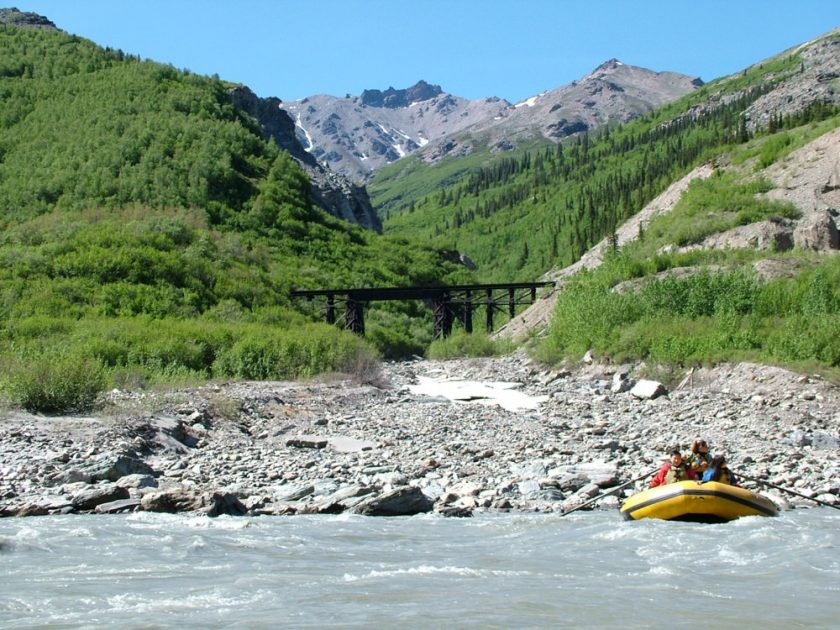The photograph captures a vibrant outdoor scene featuring a wide, bright yellow raft with three people in it, navigating a somewhat turbulent gray and silver river. The raft, equipped with oars, seems to be moving toward the viewer. The river is dotted with whitewater crests, hinting at its choppy nature. In the foreground, a rocky shoreline transitions into a valley, where a black rail bridge stretches across, supported by sturdy metal beams. On either side of the river, lush greenery with bushes, grass, and sporadic trees climbs the hillsides. The right hillside ascends sharply and is rocky with patches of evergreens, while the left side is more verdant. Beyond this lush valley, tree-covered hills give way to towering, snow-capped mountains under a clear, blue sky, creating a dramatic and scenic backdrop.